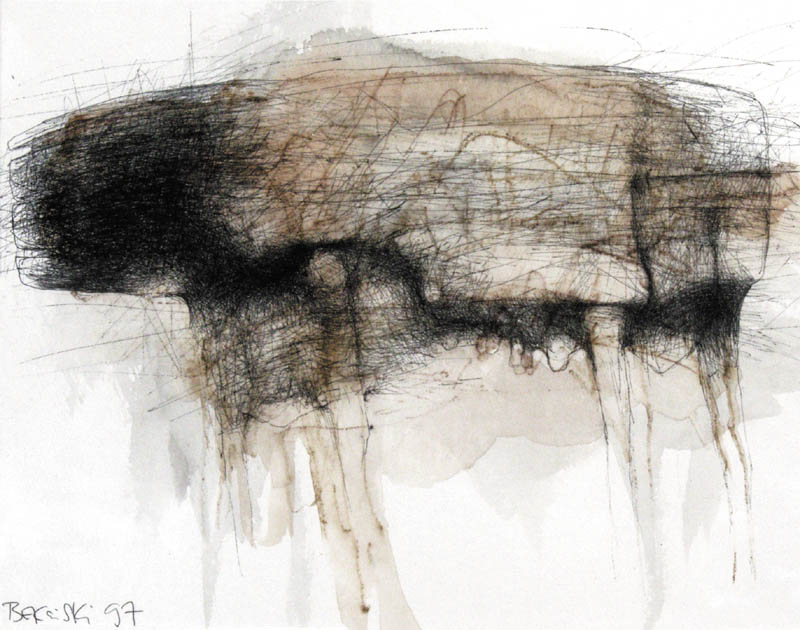The painting appears to be an abstract mixed-media depiction of a buffalo, rendered with a combination of scribbles and outlines that form a four-legged animal's silhouette. The upper portion of the image showcases a heavily scribbled black head and a light brown body interspersed with white, while the lower part reveals very thin, brown legs supporting the figure. The figure's structure is somewhat geometric, with its back side resembling a square, and black scratches permeate throughout, creating shadows and a sense of depth. The piece employs dark, thin lines and brown splotches akin to watercolor stains, imbuing it with an almost coffee-stained appearance. A light cloud formation is visible behind the buffalo against a predominantly white background, enhancing the painting's ethereal quality. An artist's signature, "B-A-C-E-S-K, 97," is inscribed in freehand black ink in the bottom left corner, with an "R" positioned at the top. The juxtaposition of deliberate shading and scribbles lends the piece an intricate and deliberate three-dimensional effect, highlighting the skill behind its creation.